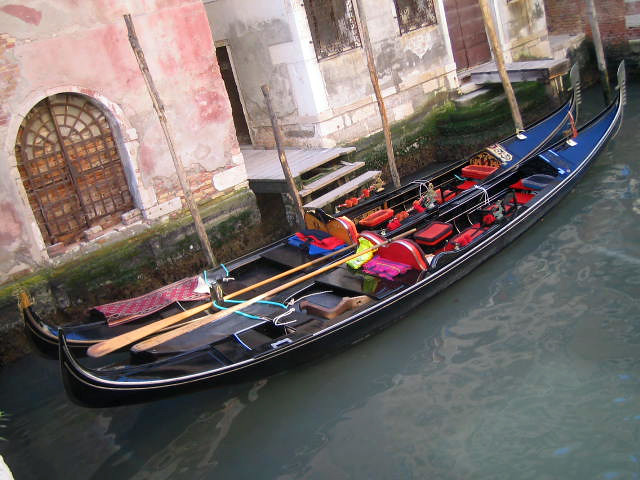This vibrant color photograph captures a picturesque scene of two docked gondolas on a murky, slate-gray canal in Venice, viewed from a bridge. The gondolas, characterized by their black and blue curved tips, house long wooden oars, red picnic baskets, blankets, and safety gear with red and white seats. They are moored by five slender, barren wooden poles protruding from the water. The tide is out, revealing green moss and seaweed clinging to the canal walls. To the sides, there is an alley between a salmon-pink building with an arched doorway and a brown security gate, and a white building with pale gray and yellow stonework, a brown door, and decorative window security fences. The intricate details of the gondolas and surrounding architecture reflect the quintessential Venetian charm.